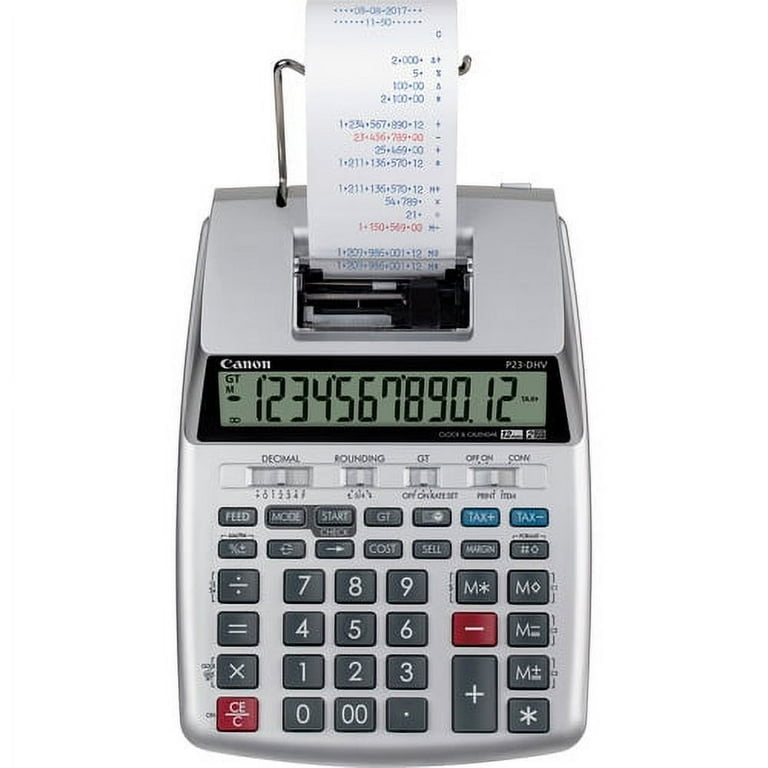This image features a detailed, close-up view of a multifunctional printing calculator by Canon, set against a white background. The device is silver with dark gray buttons, each marked by white numerals and symbols. The front panel is densely populated with standard numerical keys (0-9, including double zero), arithmetic symbols (+, -, ∗, ÷), and other specialized function keys such as decimal and rounding controls. Unique to this model, the 'Clear' and 'Subtract' buttons are distinctly red.

Above the keypad, a thin screen displays a series of lit numbers, indicating active usage. Encircling the screen is a black border, marked with the text "DT," "M," and an infinity symbol, suggesting additional multifunctional capabilities. Prominently, the Canon logo is situated in the upper left-hand corner of the screen. 

At the top of the calculator, a roll of white receipt paper is visibly loaded, feeding through a dedicated slot. The partially printed receipt protruding from the device showcases a mix of red and blue printed text, corroborating the calculator's dual-color printing feature. The machine's robust design and visible usage imply it is ideal for intensive tasks, possibly suitable for accountants or store owners managing frequent transactions.